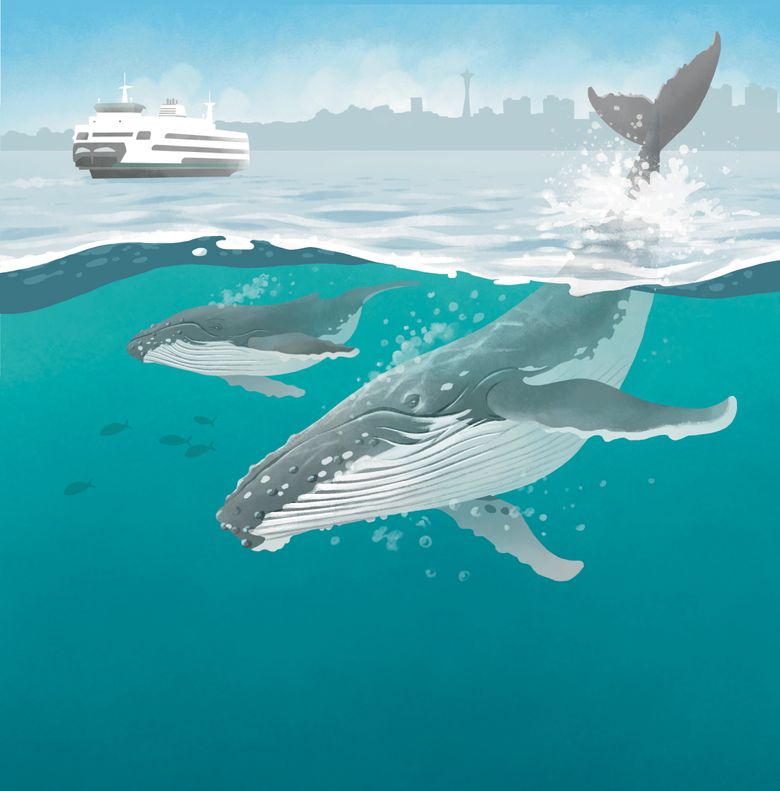This multi-colored artistic print is a vertically rectangular illustration depicting a dynamic ocean scene. The top segment of the image reflects a serene sky dotted with white clouds and a silhouette of a city skyline, possibly evoking Seattle with its recognizable needle-like structure. A large white cruise ship sits in the upper left, partially obstructed by the clouds. The majority of the piece captures an underwater vista, where the teal-tinted water is filled with life. Dominating this aquatic domain are two whales—an adult and a juvenile—gracefully diving downwards. The adult whale's tail breaches the water's surface, creating a splash above. Both whales are surrounded by air bubbles emerging from their blowholes, adding a sense of motion to the composition. Smaller fish swim nearby, enriching the scene with additional details of marine life. The contrasting shades of blue and green unify the atmospheric and underwater realms, making this piece a vivid homage to the beauty of nature.